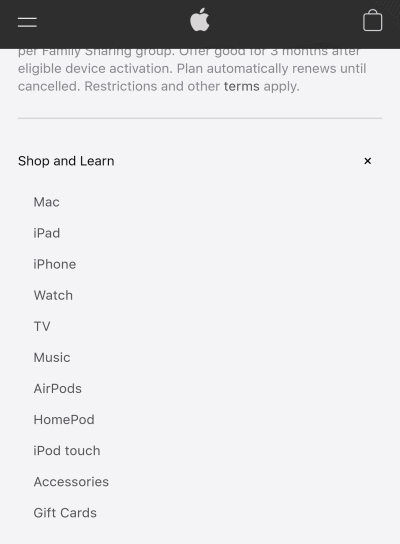The image appears to display either an iPhone or a tablet screen with a prominent user interface. At the top left, there are two horizontal lines stacked over each other, likely representing a menu icon, followed by an Apple logo. On the right side, there is an icon that resembles a shopping cart or basket. These icons are aligned beneath a black banner that stretches horizontally across the top of the screen. 

Below the banner, a message reads: "Per family sharing group, something good for three months at our eligible device activation. Plans automatically renew until canceled. Restrictions and other terms apply." Due to text truncation, only the bottom part of the first line is visible. 

Under the message, there is a section titled "Shop and Learn," followed by a vertical list of Apple product categories: Mac, iPad, iPhone, Watch, TV, Music, AirPods, HomePod, iPod Touch, Accessories, Gift Cards. All this text appears in white and is left-justified against a black background. 

On the right-hand side of "Shop and Learn," there is an X icon, likely meant for closing this section.

The overall design, including the icons and text presentation, is consistent with Apple’s design style, although there are no usual indicators of a phone's status bar (e.g., battery life, signal strength) that would confirm the device type. Therefore, the image could be from either an iPhone or a tablet.